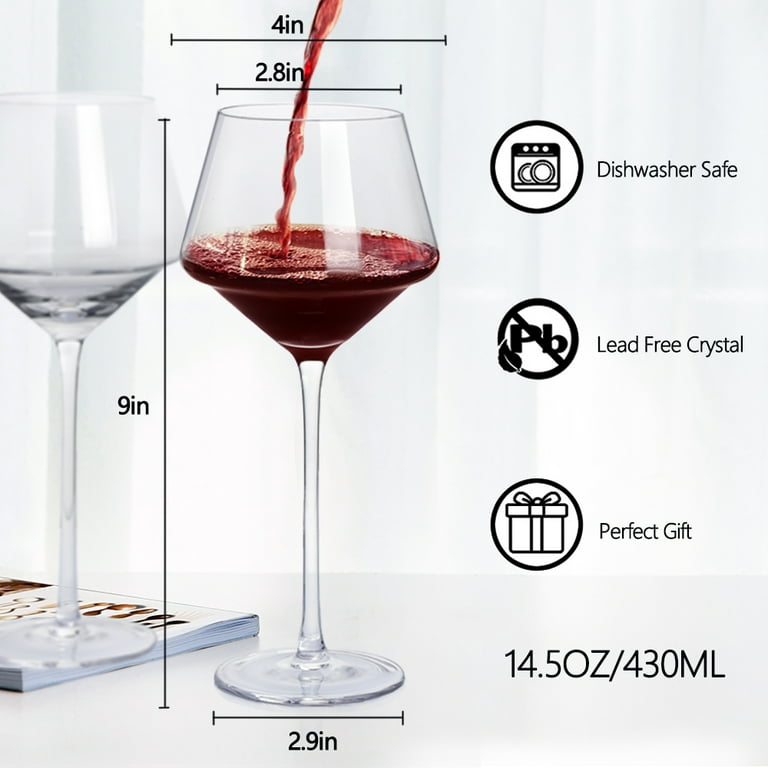The image is a detailed photograph with diagrammatic elements, showcasing two transparent wine glasses against a gray background, slightly taller than it is wide. The prominent glass, positioned slightly left of center, has grape-colored wine being poured into it, indicated by rich dark purple liquid cascading from above. This glass has various vertical and horizontal lines marking its dimensions: a vertical 9-inch line from base to top, a 4-inch horizontal line representing the widest part, a 2.8-inch line for the mouth, and a 2.9-inch line for the base diameter. The second, similar wine glass positioned to the left, is empty and reflects light off its glass surface. Both glasses have elegant long stems and circular bases, resting on what appears to be an off-white to bluish magazine or book.

To the right side of the image, three circular icons are displayed: the top icon shows a dishwasher with the label "dishwasher safe," the middle icon features "PB" with a strike-through, labeling it "lead-free crystal," and the bottom icon depicts a ribboned gift box with the label "perfect gift." The image also includes a large text indicating the capacity of the glasses as 14.50Z/430ML. This combination of photographic detail and diagrammatic dimensions emphasizes both the aesthetic and practical aspects of these wine glasses, underlining their elegance, safety, and suitability as a gift.